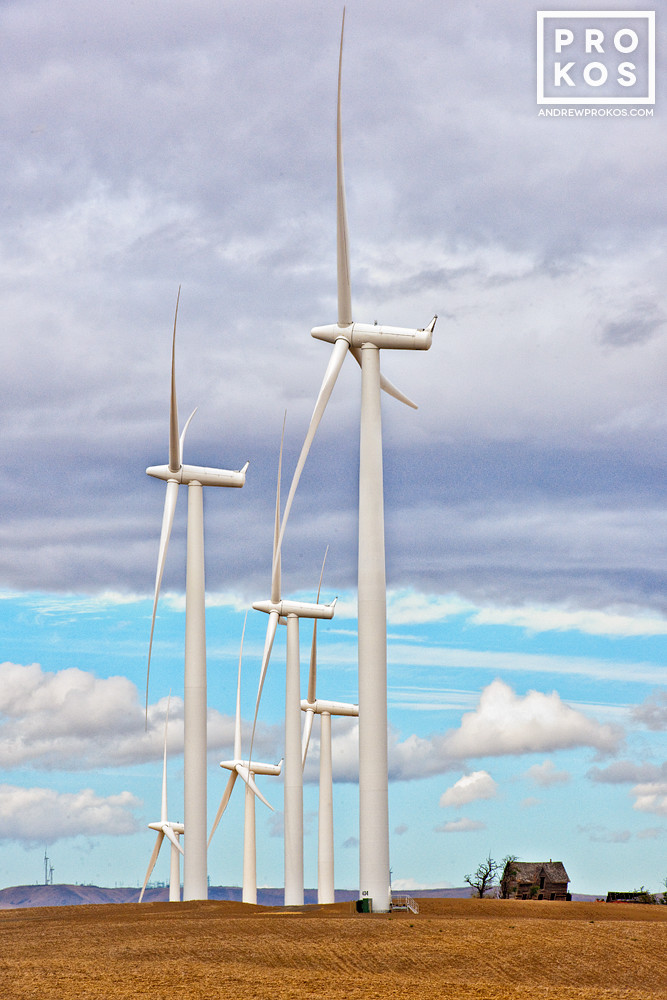This outdoor photograph captures a clear, sunny day with a horizon partially adorned with big fluffy clouds and others hinting at an approaching storm. Six tall, white windmills with three blades each dominate the center of the image, all perfectly aligned and generating electricity as they face leftward, gradually diminishing in size towards the background. The ground appears barren with patches of grasses. Off to the right in the distance, there is a dilapidated wooden building, significantly shorter compared to the towering windmills, suggesting it is about ten times smaller. A lone tree stands in front of this weathered structure. Beyond, the horizon showcases rolling hills or mountains subtly emerging from the landscape, adding a sense of depth and serenity to the composition. The image also bears a watermark in the upper right-hand corner, reading "Prokos Andrew Prokos.com".